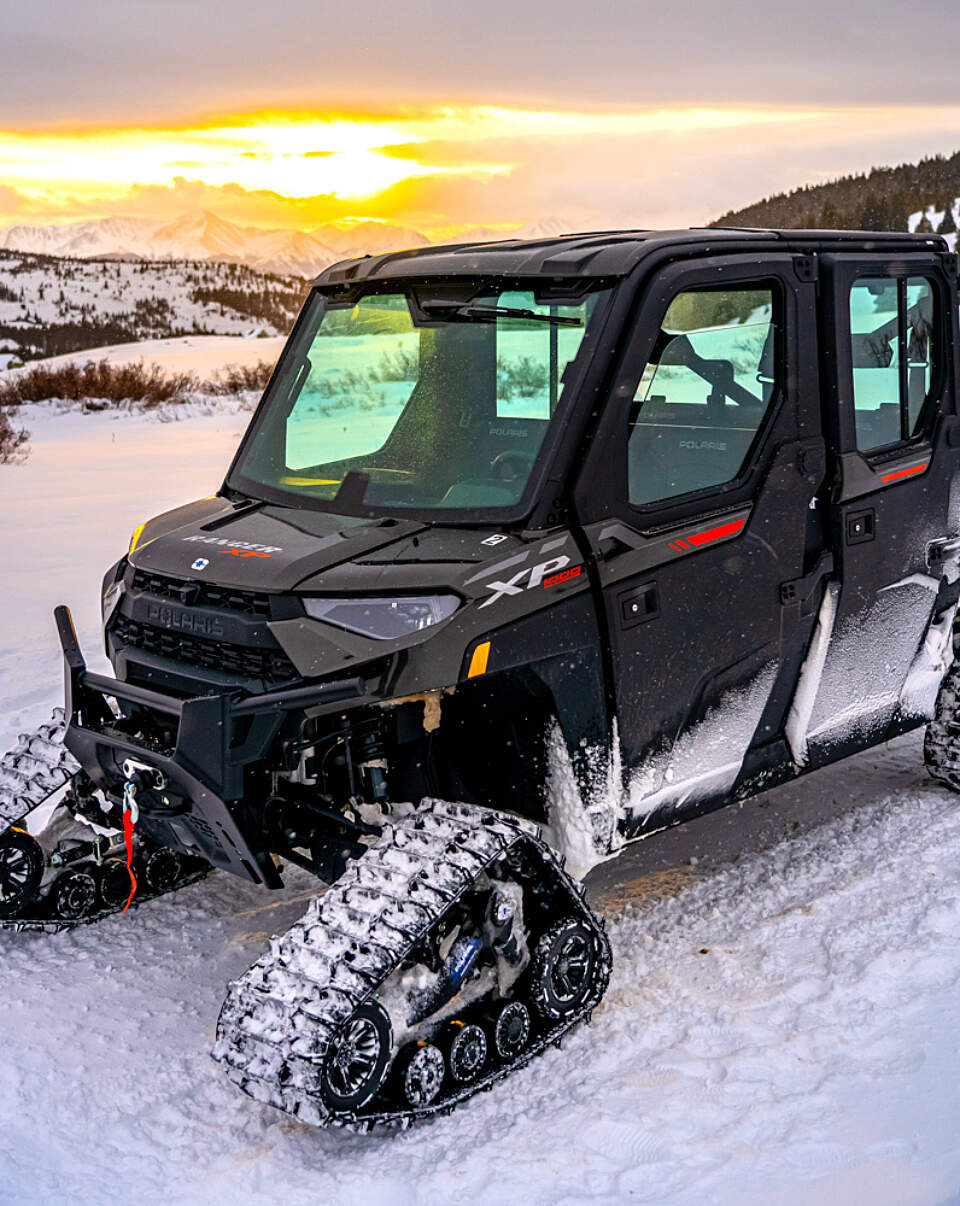The image showcases a small, modern snowmobile, prominently positioned in the center of the photograph, that has been adapted for sandy terrain. The snowmobile, which is a black Polaris model with yellow accents, features a distinctive front bull bar and a winch. The vehicle is branded with "XP" and has red accents on its right side. Instead of traditional wheels, it is equipped with specialized tracks akin to those found on a backhoe, enhancing its traction in snowy conditions. The four-door snowmobile has Polaris-branded seats visible inside. A plow connector is situated below the front grille. The setting is an outdoor snowy landscape, characterized by brown weeds poking through the terrain and scattered patches of grass. In the background, sharp, ice-capped mountains stand tall beneath a cloudy sky, with pockets of sunlight breaking through. On the far right, a dense forest of evergreen trees rises against the horizon, illuminated by the orange hues of a setting sun. The scene combines the cold, snow-covered ground with the warm, golden light from the sun, creating a striking juxtaposition between the vehicle and its surroundings.